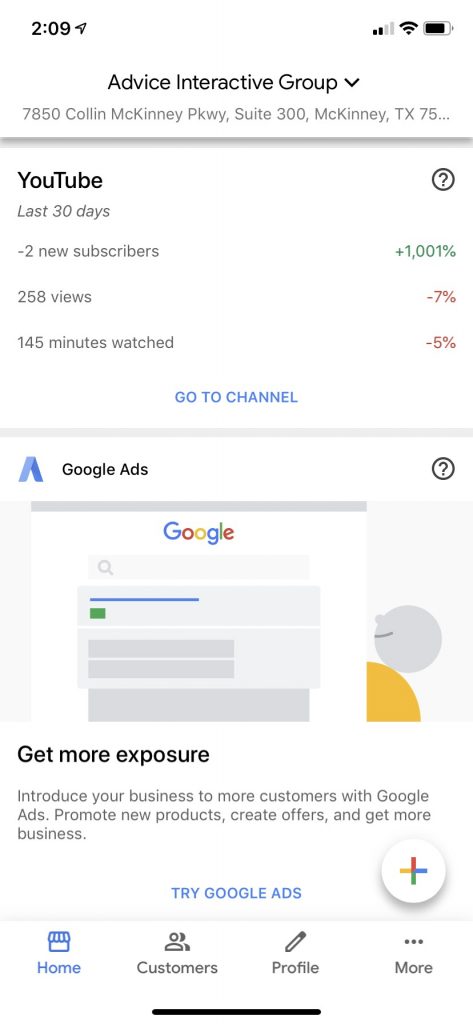**Detailed Caption:**

This image depicts a cell phone screenshot displaying the YouTube analytics dashboard for a YouTube channel named "Advice Interactive Group." The screenshot is presented on a white background with predominantly black or gray text. 

At the top left corner of the screenshot, the current time displayed on the phone is 2:09. In the top right corner, there are various icons indicating the phone's current data and Wi-Fi signal strengths, along with the battery level, which appears to be approximately 80% charged.

Centered at the top of the screen, the name "Advice Interactive Group" is prominently displayed in black text. Just below this, the physical address of the group is listed in light gray text: "7850 Collin McKinney Parkway, Suite 300 McKinney, Texas."

Further down, the screen reveals a segment of YouTube analytics specific to the last 30 days for the channel. This includes statistics on the number of gained subscribers, total views, and the aggregate minutes watched on the channel. Centrally positioned below these analytics, there is a blue hyperlinked text labeled "Go To Channel," serving as a direct link for navigating to the YouTube channel in question.

Beneath these primary analytics, there's information about Google Ads presented through a visual advertisement. The ad text encourages channel owners to "Get More Exposure" by introducing their businesses to a broader audience through Google Ads. It suggests promoting new products, creating special offers, and increasing business visibility. The advertisement's call to action is highlighted in blue text at the bottom center of the screen with the phrase "Try Google Ads."

Overall, this image provides a comprehensive insight into the key performance metrics of the "Advice Interactive Group" YouTube channel, offering a glimpse at subscriber growth, viewer engagement, and promotional opportunities through Google Ads.